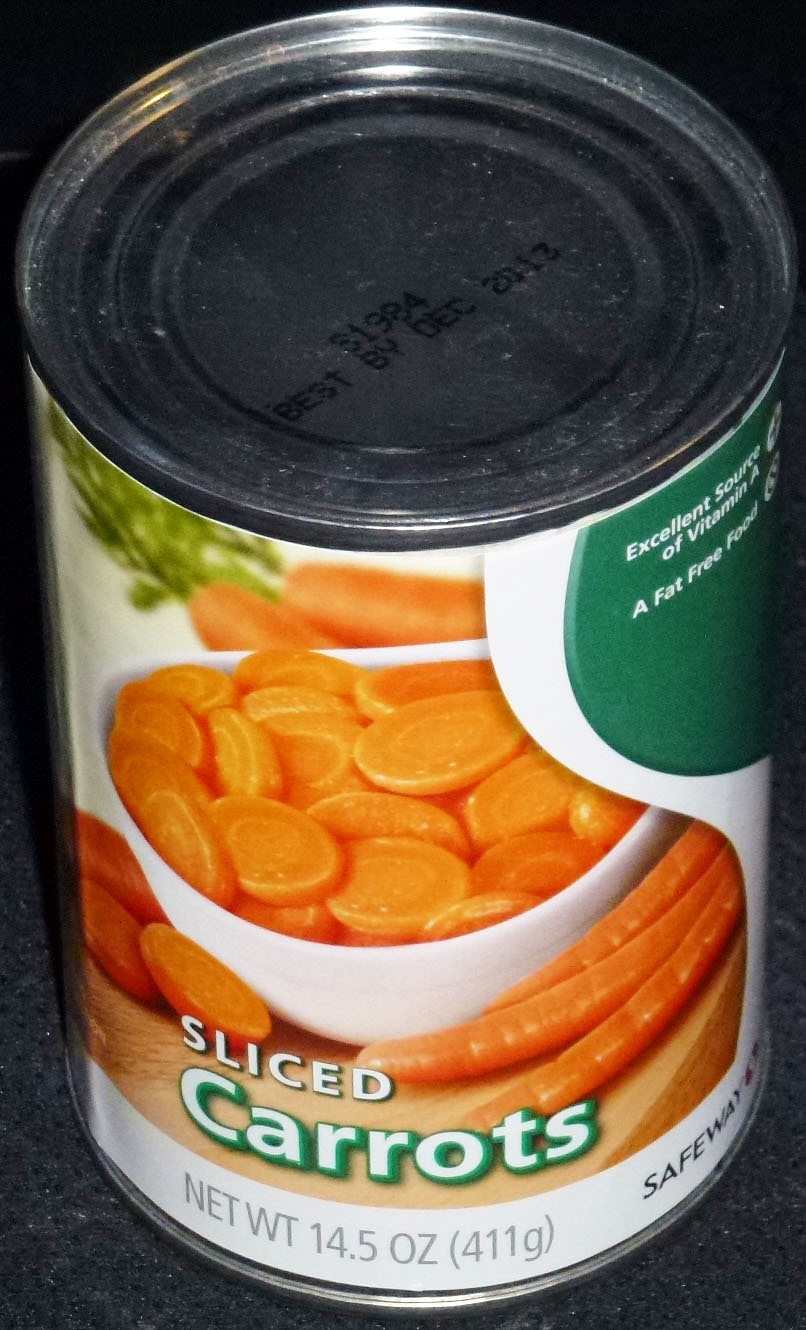The image displays a closely-cropped photograph of a tin can of Safeway brand sliced carrots. The can's label is prominently white, green, and orange. In the foreground, a white bowl brims with circular carrot slices, while additional sliced and whole carrots rest beside it on what appears to be a butcher block tabletop. "Sliced Carrots" is written in white letters with a green outline just below the bowl image. Additionally, the label states "Net Weight 14.5 ounces (411 grams)" in dark grey font underneath the product name. On the top right of the label, printed in a green background with white lettering, it reads "Excellent Source of Vitamin A" and below that, "A Fat-Free Food." The brand name "Safeway" is printed in black on the bottom right corner of the label. The metallic top of the can includes a lot stamp and a "Best by December 2013" date. The reflective nature of the metallic surface causes some glare, contributing to the overexposed appearance of the top in the photo. The background surrounding the can is a darkish grey, visible only in thin slivers due to the tight cropping of the image.